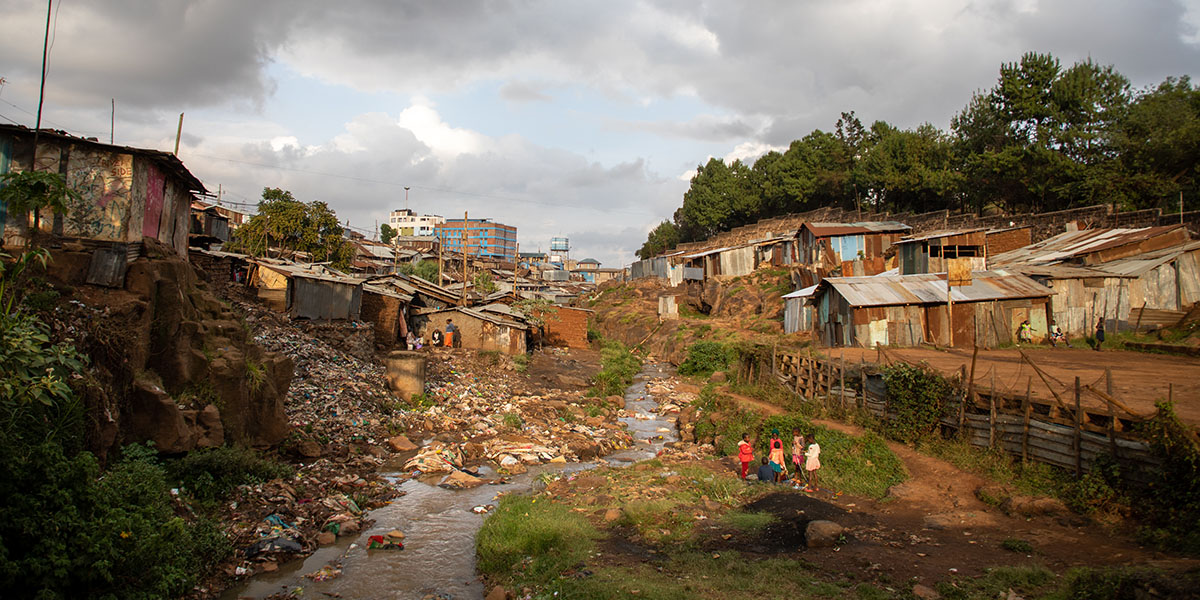This photograph depicts a slum area, likely in an Asian country, characterized by a decrepit and dirty landscape. A small, winding creek runs from the bottom left, curving right and then left, its banks reinforced haphazardly with rotting boards and steel planks. The creek is littered with garbage, and dilapidated shacks flank both sides. These shacks are constructed from rust-colored metal sheets and appear barely held together, illustrating the extreme poverty of the area. 

To the right of the creek, there is a rocky, dirt-covered expanse where a few people, including children in ragged clothes, can be seen standing and sitting. Some children are playing near the water, and a broken-down fence runs parallel to the creek on this side, dividing different levels of ground. Above the fence, the terrain is primarily dirt, extending to more rundown buildings in the background.

On the left side, the area ascends slightly into more hillside shanties, with brush and a small dirt cliff visible at the bottom. Beyond the immediate shanty town, there are more modern buildings in the far distance. The sky above is mostly overcast with gray clouds, allowing a sliver of light blue to peek through, adding a somber tone to the desolate scene.